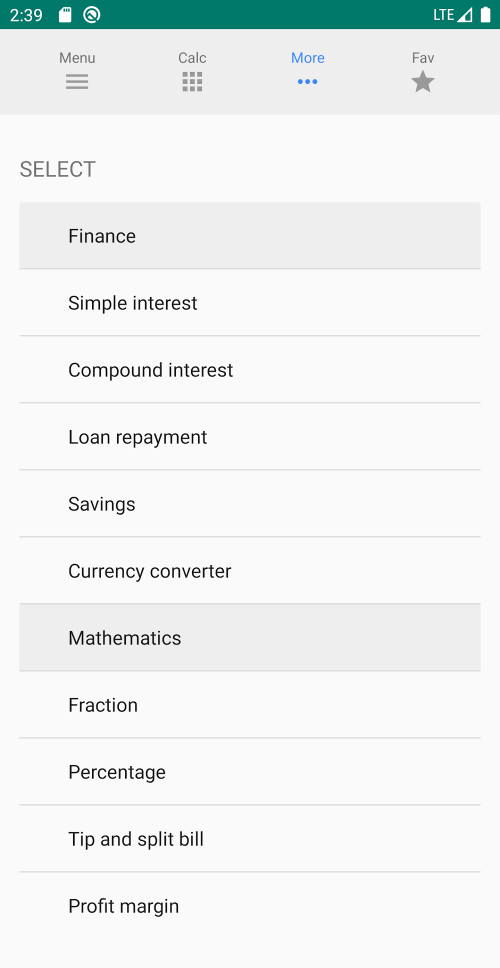The image showcases a screenshot of a financial calculator app on a device with a minimalist, white background. At the top of the screen, the current time is displayed as 2:39. Adjacent to the time, there is a menu icon represented by three horizontal lines. Below this, a horizontal navigation menu is visible, comprising four options: 

1. **Calc** - symbolized by a grid of nine squares arranged in three rows and three columns.
2. **More** - indicated by the text and an icon of three vertically aligned dots.
3. **Finance** - currently selected and highlighted in gray, featuring a list of options such as:
   - Simple Interest
   - Compound Interest
   - Loan Repayment
   - Savings
   - Currency Converter.
4. **Mathematics** - also highlighted in gray, showing options for:
   - Fraction
   - Percentage
   - Tip and Split Bill
   - Profit Margin.

Additionally, there is a subtle fade effect incorporated with a star icon to enhance the visual appeal. The layout is horizontal, offering users a clean and intuitive interface for navigating through various financial and mathematical tools.